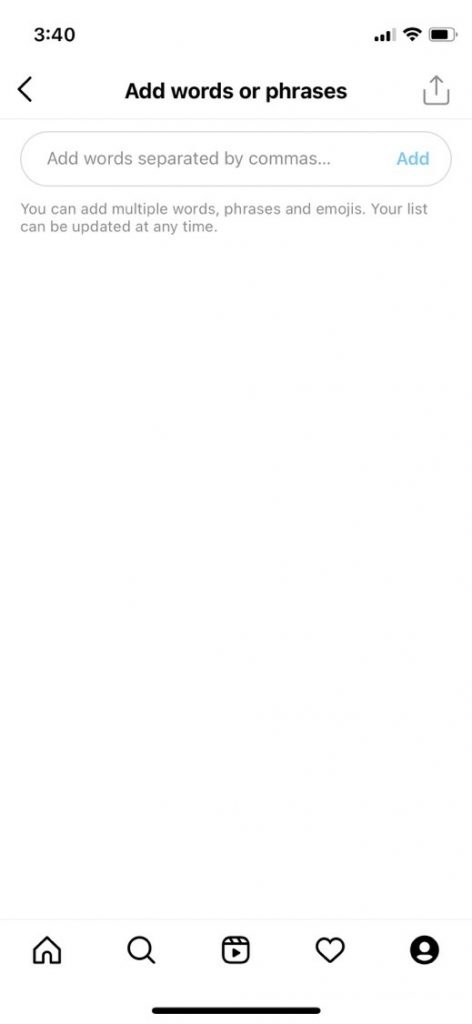The screenshot displays a phone interface with a white background. At the very top left corner, the time reads "3:40." On the top right, there are three out of four bars for cellular signal strength, a full Wi-Fi signal, and a battery icon showing approximately 75% charge.

Just below the status icons, on the left side, there is a back arrow. In the center, bold text reads "Add words or phrases." To the right, there is a forward icon featuring an upward-pointing arrow and a small staple-like symbol beneath it.

Directly below, there is a search bar or input box with placeholder text that says "Add words separated by commas." Inside this, a blue hyperlink labeled "Add." Following this, a message notifies users: "You can add multiple words, phrases, and emojis. Your list can be updated at any time."

At the bottom of the screen, a navigation bar features five icons: a house (home), a magnifying glass (search), a box with a play button inside (media), a heart (favorites), and a person icon (profile). A small black horizontal line is visible below these icons.